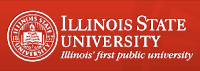The logo for Illinois State University is featured in a burgundy red rectangular box. Prominently displayed within the logo is the university's seal, which showcases an open book at its center—a symbol of learning and education. The text "ILLINOIS STATE UNIVERSITY" appears in bold, capital letters, emphasizing the institution's name. Below this, in a smaller, italicized font, are the words "Illinois' First Public University," highlighting its historical significance. This logo effectively combines elements that represent the university's heritage and commitment to education.